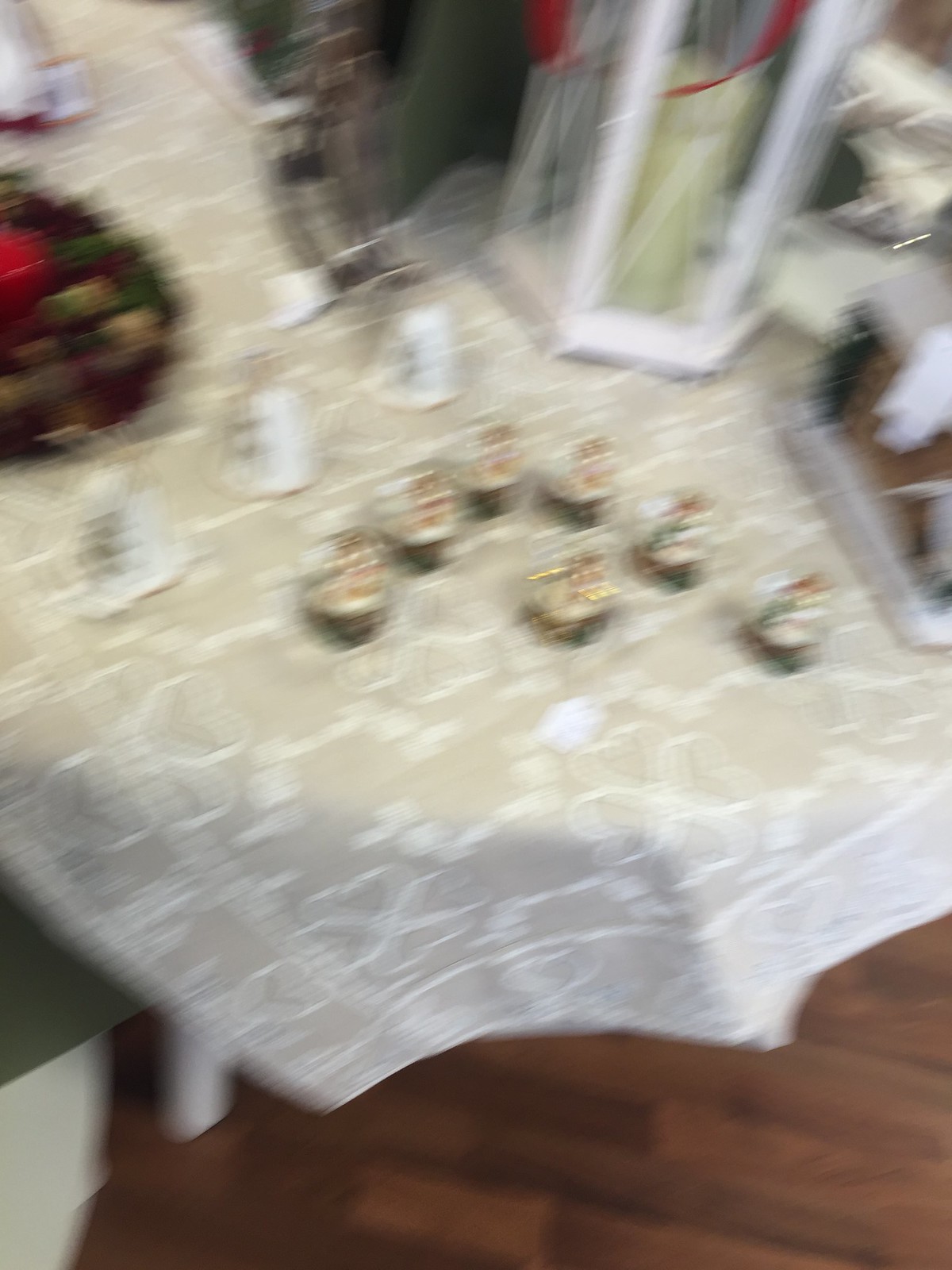In this blurry photograph taken at a downward angle, the viewer gets a glimpse of a table covered with a light beige, off-white tablecloth adorned with a delicate lace pattern featuring floral or heart motifs. The table is cluttered with a variety of items, including some small objects at the bottom and larger objects or containers towards the top, potentially suggesting an assortment of jewelry or other personal items. The camera motion during the shot results in a lack of clarity, making it difficult to identify individual items. The edge of the image reveals a dark wooden floor beneath the table, adding a contrasting background to the scene.